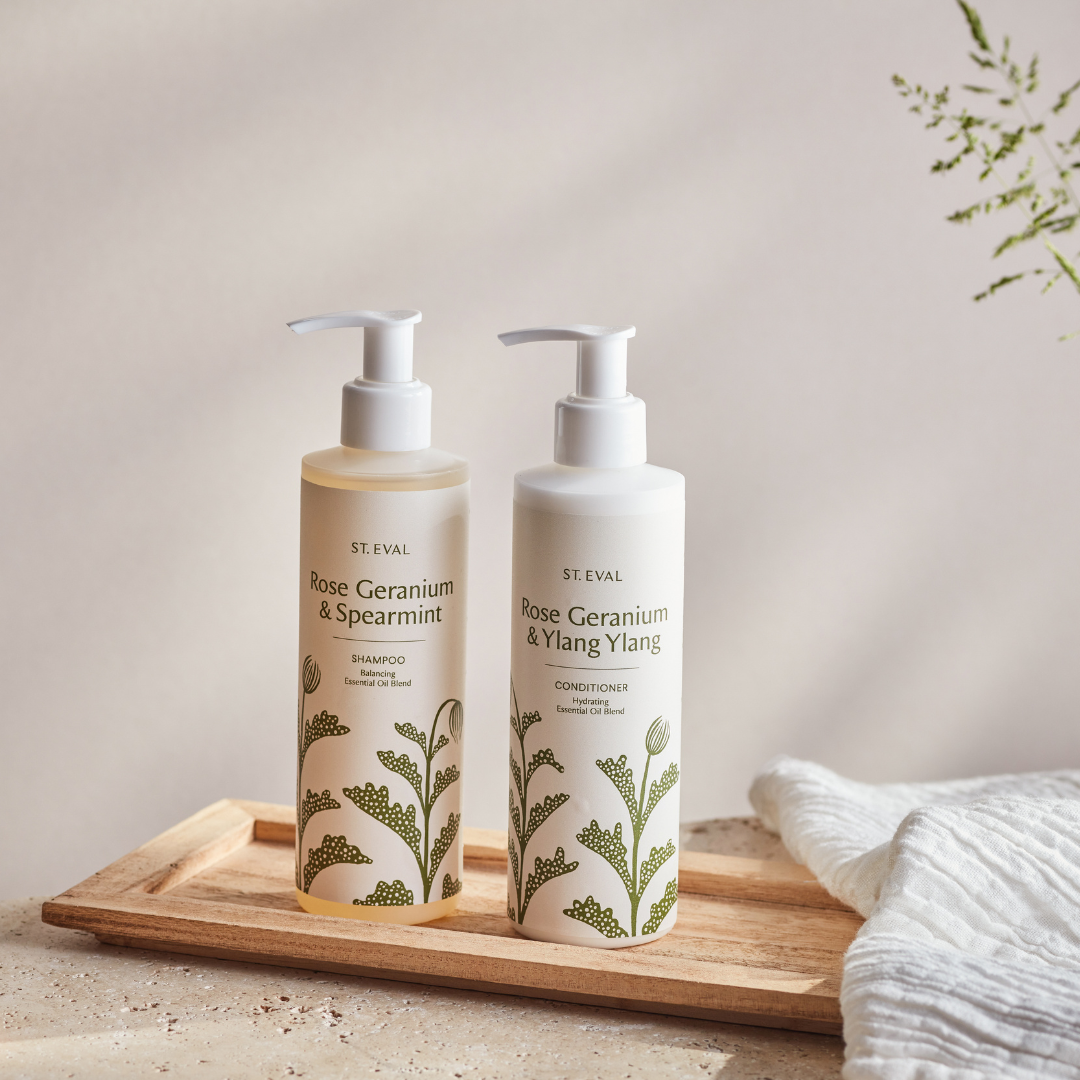In the image, set against a grayish background partially filled with small plant leaves in the top right corner, there is a light wood bamboo tray placed on a creamy, porous rock-like surface. Resting atop the tray are two white pump bottles with clear plastic bottoms. The bottle on the left, labeled "Saint E.V.A.L. Rose Geranium, Geranium, and Spearmint Shampoo," features green text and a plant illustration. The bottle on the right reads "St. E.V.A.L. Rose Geranium and Ylang Ylang Conditioner," also with green text and a floral design. To the right of the tray, partially draped over it, is a white waffle weave cloth. The overall setting includes the textured rock surface below and the gray wall behind, enhancing the natural and serene aesthetic of the composition.